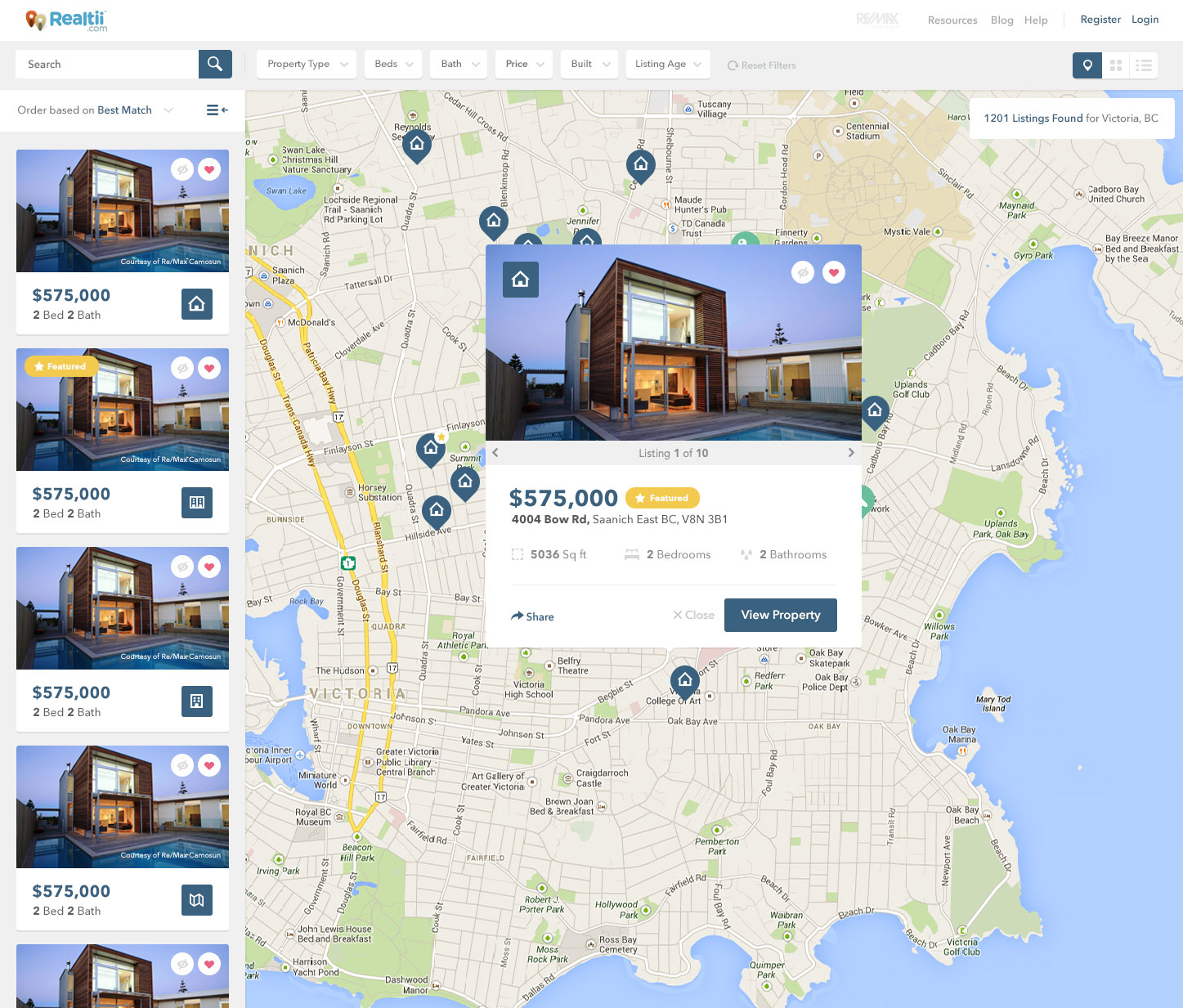A screenshot from a real estate listing website named "RealTil" (or possibly "RealT"). The interface features an empty search box at the top, suggesting that the user can search for specific homes or properties. Below the search box, the screen displays a map overlaid with numerous blue pins indicating various locations or amenities such as nearby stores like CVS.

The central focus of the listing is a modern, two-story condo characterized by its extensive glass frontage. Both the top and bottom floors feature large windows that almost entirely cover the front of the building, providing a sleek, contemporary appearance. The image hints at its urban setting, potentially adjacent to a structure that could be a hotel, although it's unclear due to image quality.

A label on the interface indicates that this is listing 1 of 10, implying there are 10 similar properties available on the market. Each condo is priced at $575,000. Additionally, the listing specifies that this particular property is located in South Carolina.